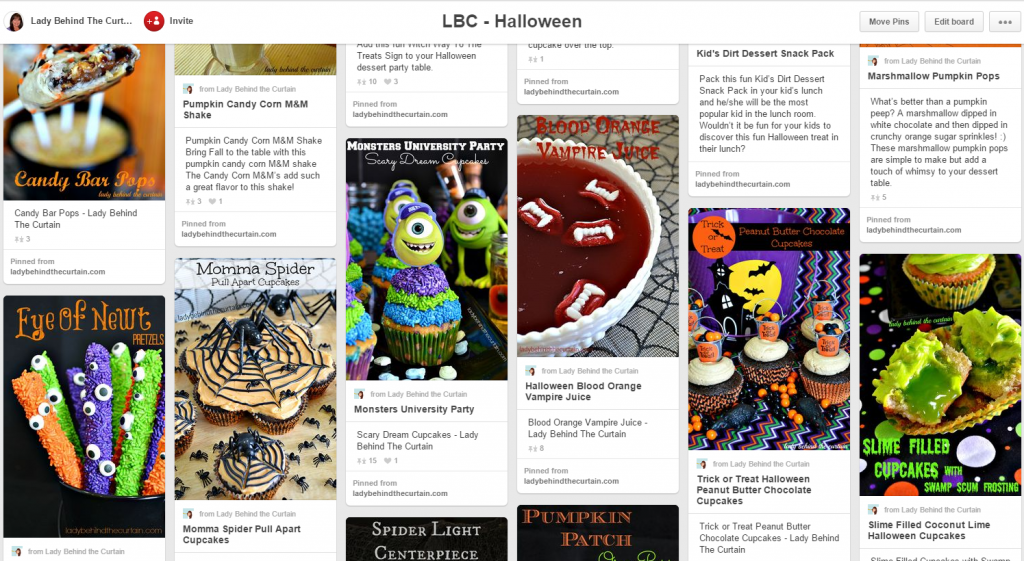The image features a festive theme titled "LBC Halloween" written in black text at the top. To the left of the title, there is a prominent red "Invite" button. Adjacent to this is the username "lady behind the cat." On the top right, three additional buttons are visible: "Move Pins," "Edit," and "Option."

Directly below, the description highlights "Marshmallow Pumpkin Pops" accented with fun details: "What's better than a pumpkin pop? A marshmallow dipped in white chocolate and then rolled in crunchy orange sugar sprinkles. These whimsical treats are simple to make and perfect for any dessert table."

The lower section of the image introduces "Slime Filled Cupcakes," featuring cupcakes filled with vibrant green slime. To the left, "Trick or Treat Peanut Butter Chocolate Cupcakes" are described as scrumptious Halloween-themed cakes with a delightful mixture of peanut butter and chocolate.

Central to the display are "Master University Party Cupcakes," each adorned with characters from Master University, and accompanied by "Halloween Blood Orange Vampire Juice," a striking red beverage. Other whimsical treats include "Pumpkin Candy Corn M&M Shakes," "Mama Spider Pull-Apart Cupcakes" topped with a black spider, "I Own You Tea Petals," "Candy Bar So Purple," a "Spider Light Centerpiece," and a playful "Pumpkin Patch" at the bottom.